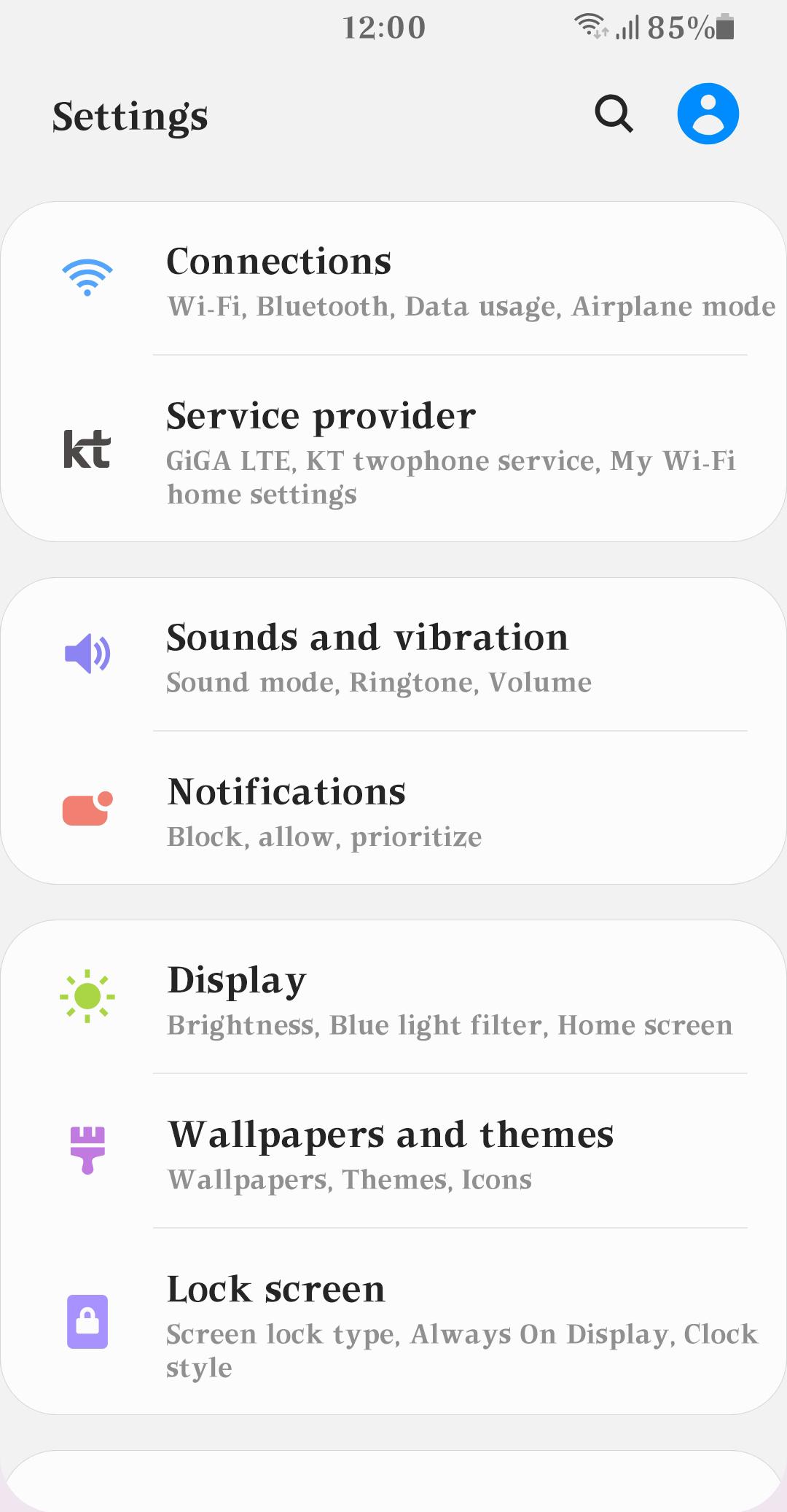The image depicts a phone settings screen with various icons and text. At the top right corner, there's an icon, and to its left, a magnifying glass indicates a search bar. The title "Settings" is displayed in a slightly irregular font. The device's status bar at the very top shows the time as 12:00. Towards the top right of this status bar, there is a Wi-Fi symbol with an 'X' beside it, indicating no connection. Adjacent symbols show four bars of 4G network signal and an 85% battery life indicator.

Below this status bar, the screen displays an array of settings options. The first section is labeled "Connections," accompanied by a blue Wi-Fi icon. This section includes options such as Wi-Fi, Bluetooth, Data Usage, and Airplane Mode, each with gray subtext descriptions. It also lists service providers like LTE and KTT, as well as individual settings for "Giggle" and specific Wi-Fi network names. Additional details include "Samsung Vibration" settings.

Continuing downward, there are several settings categories: 
- "Notifications," marked with a red notification icon.
- "Display," paired with a green sun icon.
- "Wallpapers and Themes," indicated by a purple paintbrush icon.
- "Lock Screen," which features a blue lock icon.

Each category has detailed sub-options easily accessible for the user. The layout emphasizes organized sections for ease of navigation through the phone's settings.